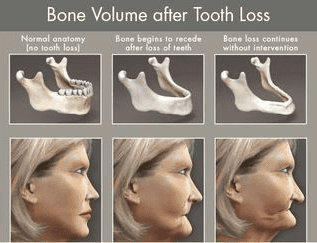The image is an educational graphic titled "Bone Volume After Tooth Loss," featuring a detailed instructional chart with three sections. Each section includes both a digital rendering of a woman's face and corresponding illustrations of her jaw and bone structure over time. The first section depicts a woman with a normal facial structure, accompanied by an illustration of a jaw with intact teeth, labeled "Normal Anatomy, No Tooth Loss." The second section shows slight jaw recession and a sunken chin, with an illustration of a jaw without teeth, annotated "Bone Begins to Recede After Loss of Teeth." The final section presents a heavily atrophied, sunken facial appearance, with an illustration showing significant bone loss in the jaw, labeled "Bone Loss Continues Without Intervention." This detailed comparison highlights the progressive impact of tooth loss on bone volume and facial structure.